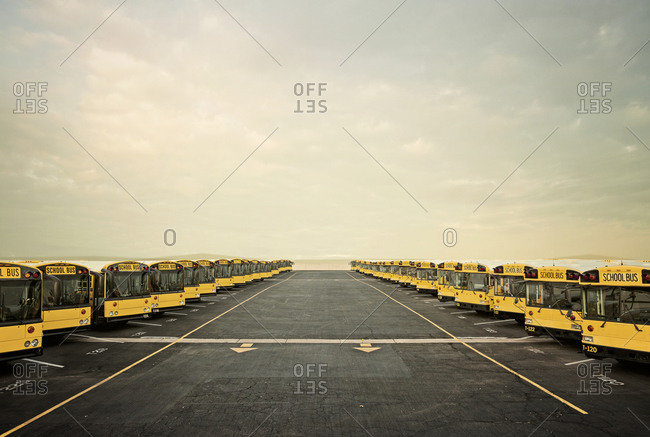In this image, we see a wide asphalt-covered parking lot filled with rows of yellow school buses parked diagonally on both the left and right sides. The buses, which feature black and yellow writing and white roofs, extend into the distance, creating symmetrical lines that draw the eye toward the horizon. Each bus has 'SCHOOL BUS' written in black letters on a yellow background across the top. The bumper of one bus visible in the foreground reads "I-20" and another has an undecipherable code. Overlaying the entire scene is a grid of diamond shapes formed by thin gray lines, with the words "OFF" and "SET" repeatedly appearing in the corners of these shapes, 'SET' notably being upside down. The ground is marked with white lines designating parking spaces, and faded numbers. The sky occupies more than half of the image, appearing mostly gray and overcast with hints of blue in the top left corner, suggesting a cold, foggy day. Yellow arrows on the asphalt direct traffic towards the front of the image. The combination of the parked buses, directional arrows, and sky creates a structured yet open scene, clearly captured outdoors.